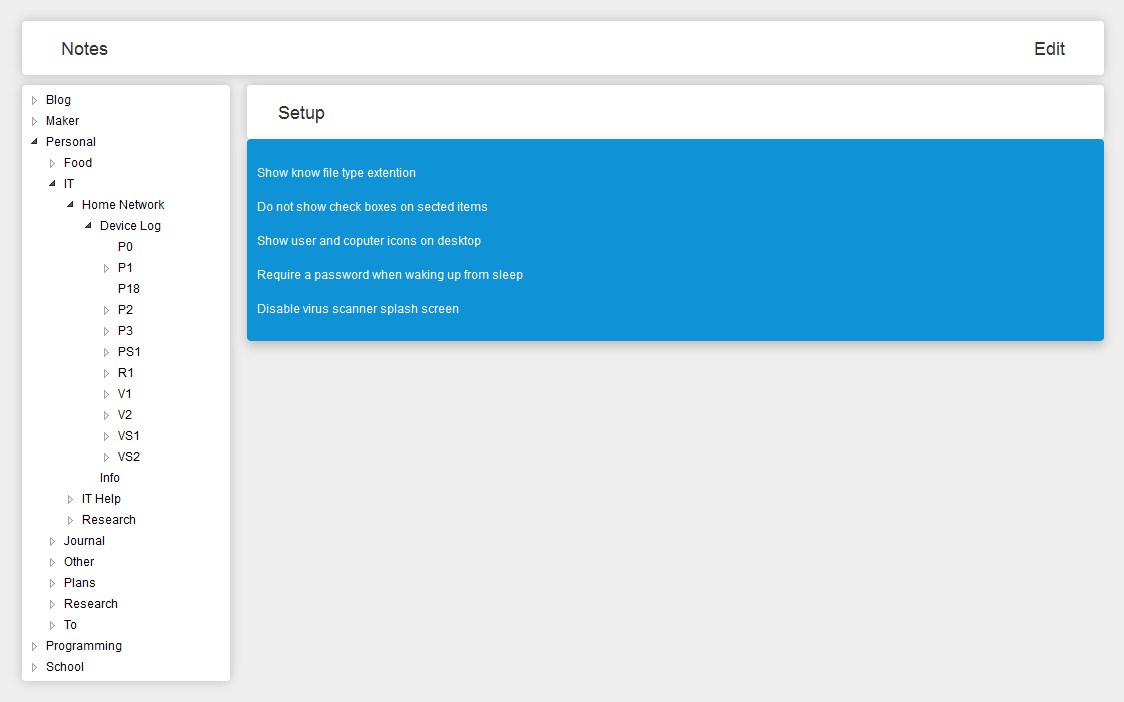A cropped screenshot displays a notes panel within a productivity suite against a gray background. A long rectangular header bar spans the top of the image, with "Notes" prominently displayed in large black font on the left side and a small black "Edit" button on the far right. On the left side of the screenshot, a white vertical box lists various categories, each with a right-pointing arrow for expanding to subcategories. The categories listed are: "Blog," "Maker," and "Personal." The "Personal" category is expanded to reveal subcategories including "Food," "IT," "Home Network," "Device Log," and further subcategories under "IT Help" and "Research." 

To the right, a large white box contains the word "Setup" in bold black letters. Below, several configuration options are listed: "Show no file type extension," "Do not show check boxes on selected items," "Show user and computer icons on desktop," "Require a password when waking up from sleep," and "Disable virus scanner splash screen," with these options highlighted within a large blue box. The lower half of the screenshot shows a blank gray area, offering no additional visual information.